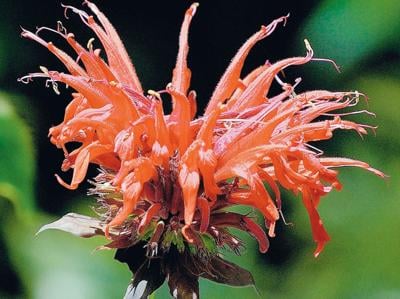This image, captured outdoors in bright daylight, prominently features a close-up of a single plant with a striking floral bloom. The flower, viewed from the side, displays multiple, thin, and somewhat messy petals that radiate outward in an anemone pattern, giving it a dynamic and textured appearance. The petals are orange with hints of pink, adorned with delicate white filaments at their tips. Beneath the large flower top, a cluster of small, vibrant green leaves peeks out from the stem, which extends downwards but is cut off at the bottom edge of the image. The background is composed of darker shadows with green highlights from blurred vegetation, adding depth and contrast to the photograph. The overall capture, in landscape orientation, emphasizes the intricate details of the bloom while maintaining a realistic and representational style.